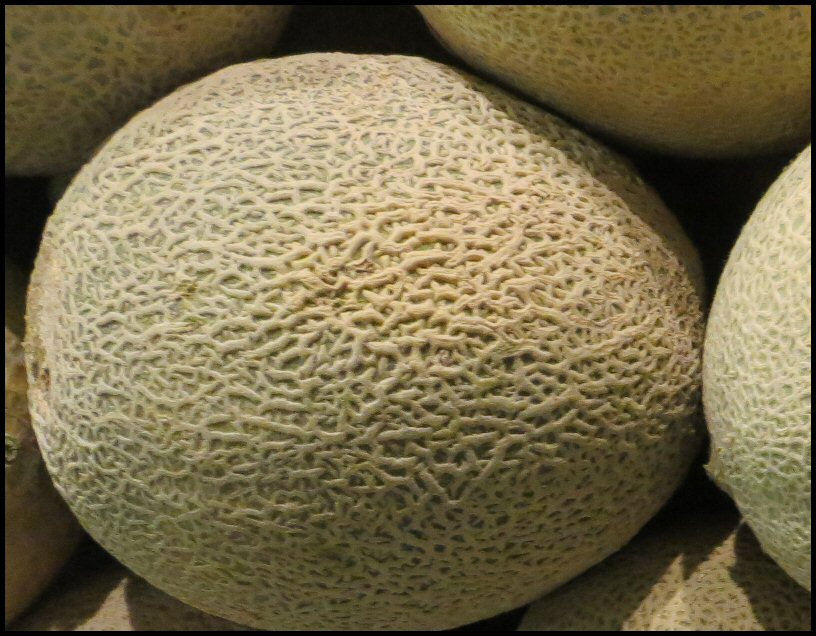The image is a color photograph presented in landscape format, featuring a close-up of a cantaloupe melon positioned prominently at the center of the frame. The main cantaloupe showcases a distinctive textured rind with a webbed pattern of shallow, crisscrossing grooves and a combination of greenish undertones and brown tinges on the right side. Additionally, there are indications of a yellow spot likely from where it rested on the ground during ripening. Surrounding the main cantaloupe, partially visible melons can be seen, suggesting they are in a bin or crate, much like one would find in a grocery store. The overall lighting is even, possibly indicating an indoor setting with artificial light. Shadows create interesting shapes between the melons, with triangular pockets forming where they meet, and a thin black line outlines the entire image. The photograph captures the ripe, textured surface of the central melon, highlighting it against the slightly out-of-focus background melons, each adding depth and context to the scene.